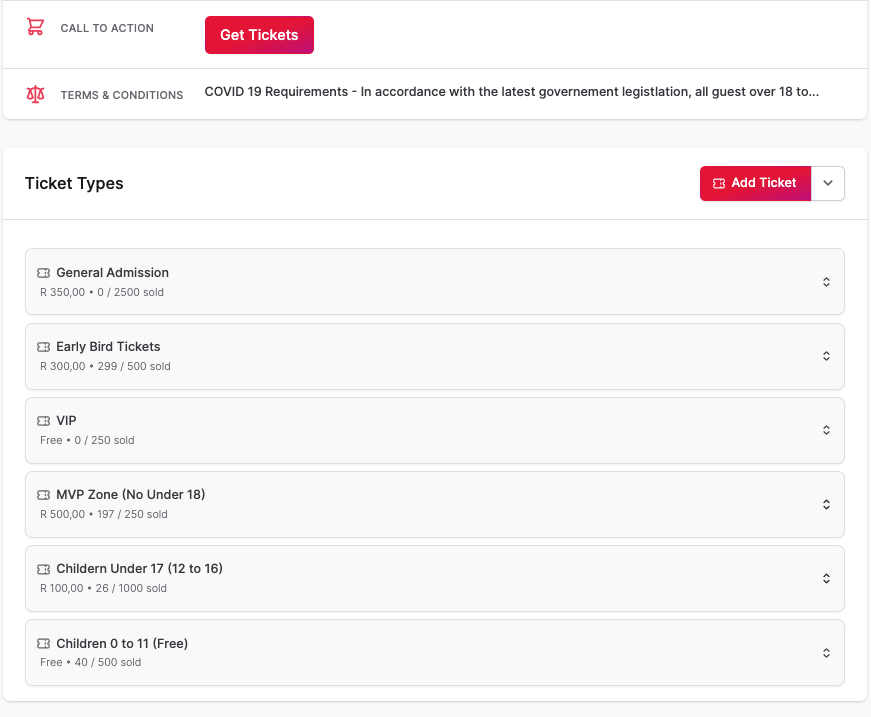This screenshot captures a ticket sales website interface. In the upper left-hand corner, there is a red shopping cart icon. Adjacent to the right, there is text reading "Call to Action," followed by a prominent red button with white text that says "Get Tickets." Below this, on the left side, an icon representing scales is shown, next to the label "Terms and Conditions." It is also noted that there are specific COVID-19 requirements in accordance with the latest government legislation, with a mention that all guests over the age of 18 must adhere to these guidelines. 

Further down the page, there is a section dedicated to various ticket type options. On the right side of each option, a red "Add Ticket" button with white text is present. The ticket types are listed in a vertical format and include several categories: General Admission, Early Bird Tickets, VIP, MVP Zone, No Under 18, Children Under 17, Ages 12 to 16, and Children Ages 0 to 11 (free admission). 

This website layout provides a clear and organized way for users to navigate ticket purchasing, complete with highlighted call-to-action buttons and detailed ticket type categorization.